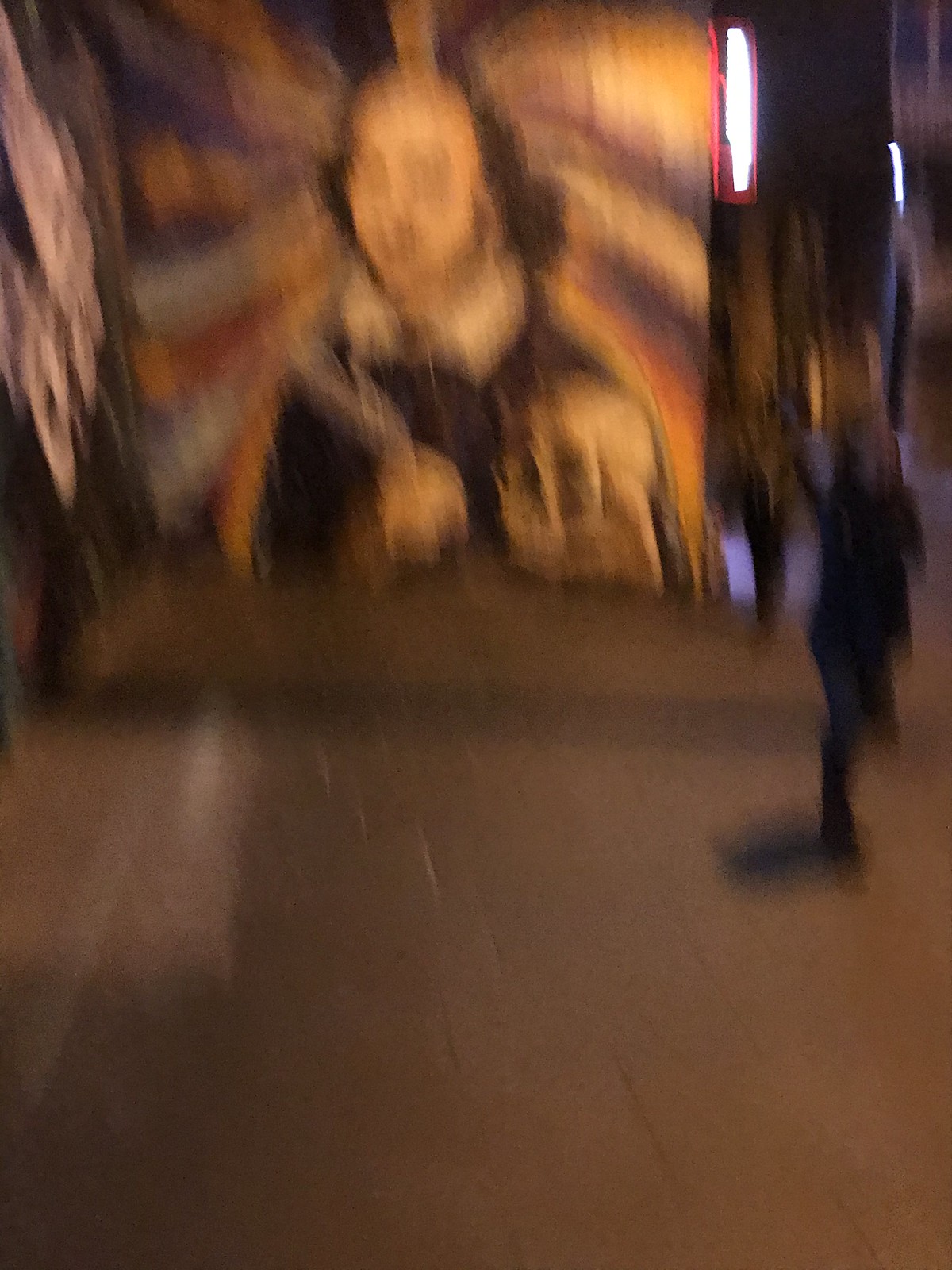This color photograph, captured in portrait orientation, presents a scene that is somewhat blurred, making it challenging to discern specific details. The foreground features a wooden brown floor, giving the image a warm and rustic feel. Dominating the back wall is a large, floor-to-ceiling painting depicting a man. The man, dressed in a white shirt with a white collar and what appears to be a black sweater or coat over it, holds a feather quill in one hand, while the contents of the other hand remain indistinguishable. The backdrop of the painting is a mix of dark brown, golden, beige, and intermingled purple hues, adding a rich complexity to the scene.

In the immediate foreground is a person walking toward the viewer, identifiable by their boots, blue jeans, and a long black coat. To the side, a few papers are affixed to the wall, adding to the environment's textured layers. Further back, beyond the approaching figure, there's another hallway leading to an open doorway through which light streams in, casting a gentle illumination into the space.